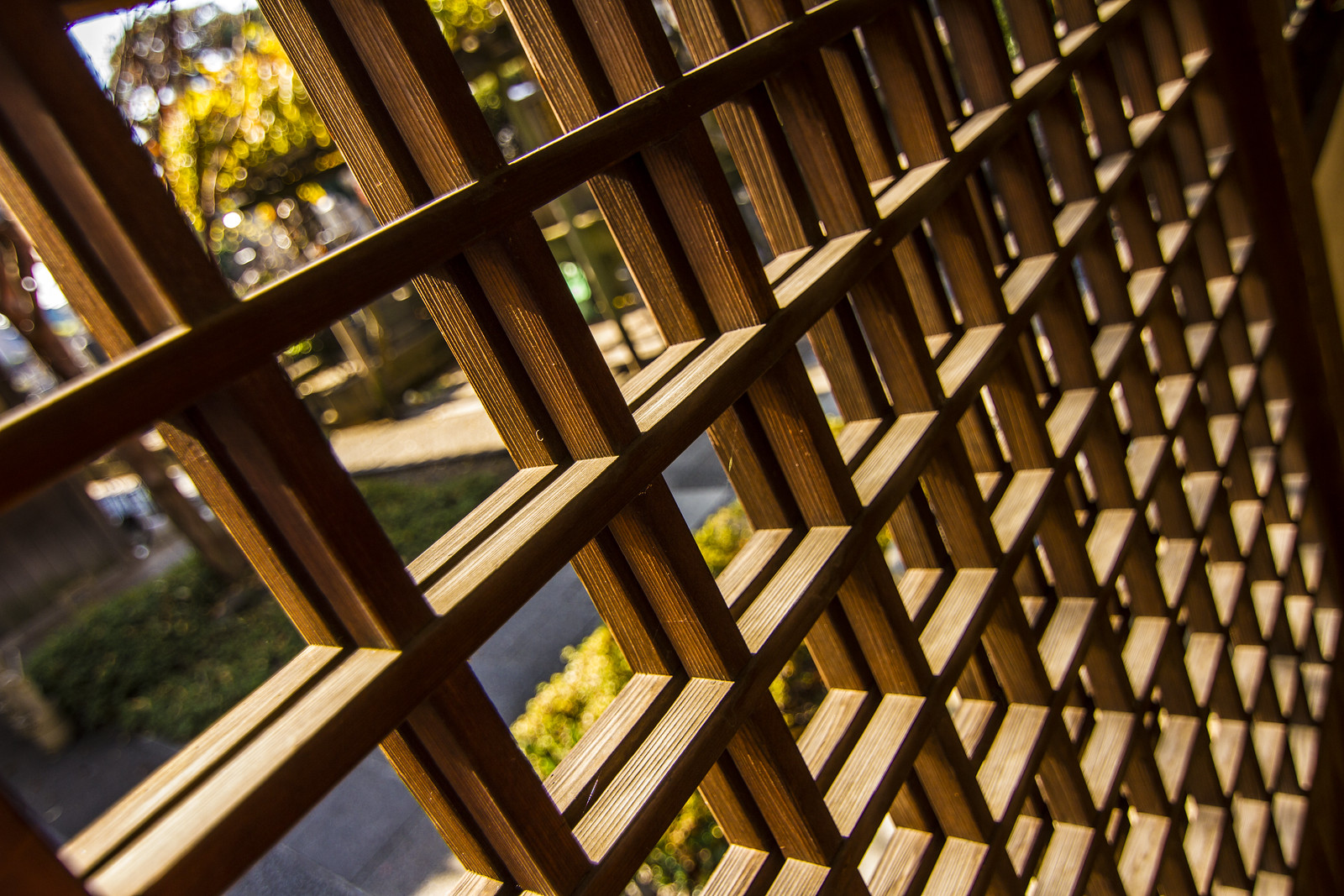The photograph captures an outdoor scene viewed through a large wooden grid, possibly a wooden gate or grate, which covers a window without glass. The wooden structure, composed of uniform square patterns, is light brown with varying tones of darker brown and black, giving it a well-crafted but unvarnished look. This grid angles diagonally from the top left to the bottom right of the image. The outdoor view seen through the grid is slightly blurry but reveals a bright, sunny day reminiscent of Southern California. The yard outside is well-maintained, featuring a bush, a stone or concrete walkway, green grass, and several trees. In the far distance, a light green object is visible but indistinguishable. The overall symmetry and craftsmanship of the wooden grid frame the sunny, serene outdoor scene perfectly.